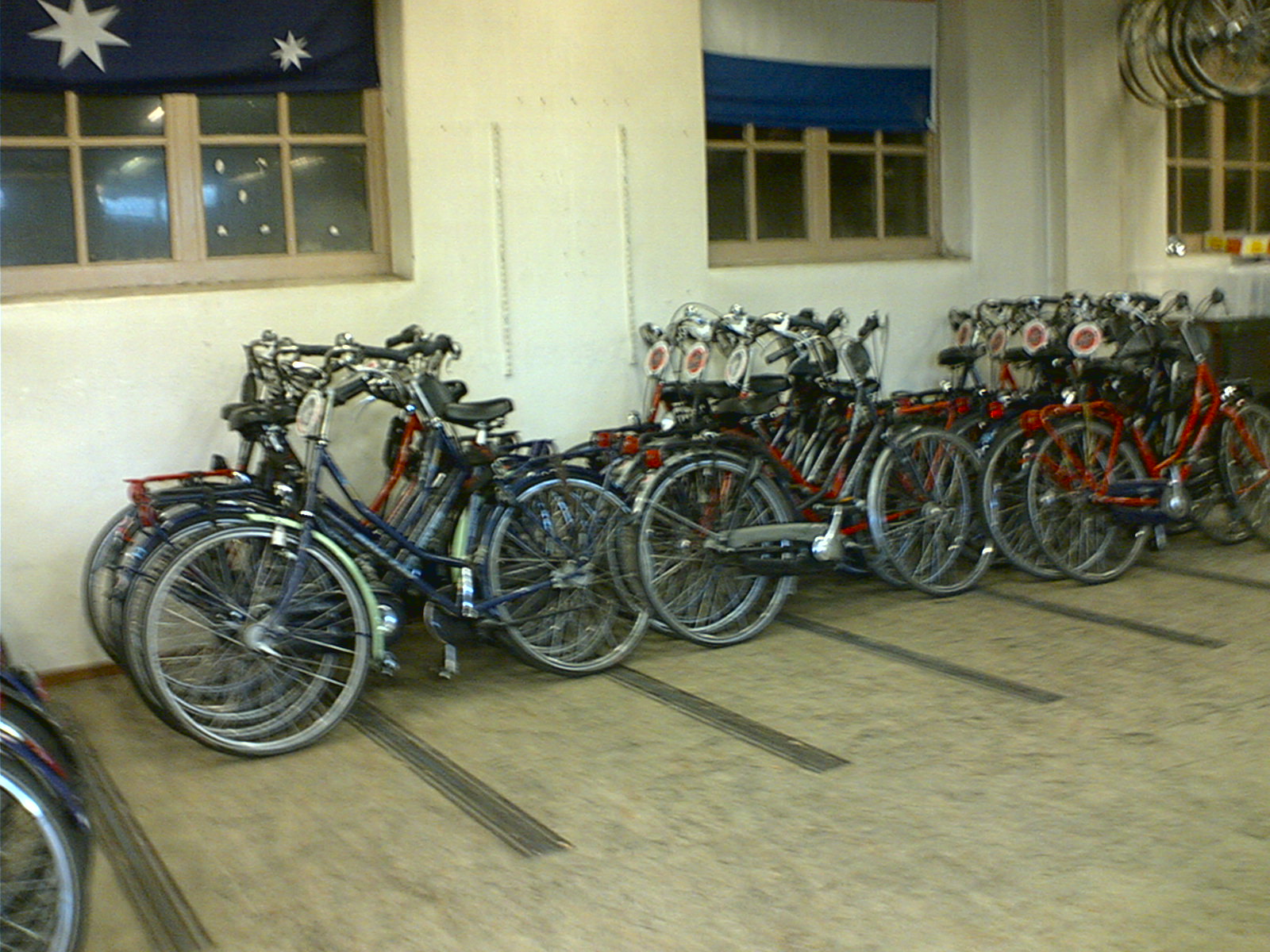The picture showcases the interior of a bustling bicycle shop with a polished hardwood floor. Lining the back wall, which is painted white, are two windows; the left window features a blue and white flag with white stars, while the right window sports a blue and white shade with a star motif. A third window is visible, partially obscured by bicycles hanging closer to the ceiling. The shop floor is organized with rows of bicycles, approximately 12 to 15 in total, predominantly red and blue with metallic trim and some adorned with a flower symbol on the front. These bicycles, arranged in at least three rows, have various designs catering to both younger individuals and adults. The back left row and middle row are mostly red bicycles, while the front row displays a mix of two blue and one red bicycle. Additionally, several bikes in the upper corners and scattered wheels near the bottom right further fill the space, along with some bicycles equipped with rear racks for carrying items.